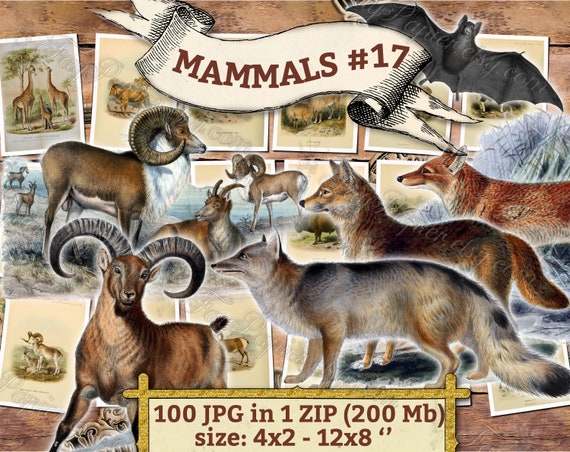The image titled "Mammals Number 17" showcases a diverse collage of mammal illustrations layered throughout. Dominating the upper right is a black bat with a small white patch around its muzzle. Situated below the bat is a red fox, followed by a brown fox slightly forward and a gray winter fox beneath them. The left side of the image features a series of ram illustrations; a central brown ram, another ram above it, a smaller ram to the right, and an even smaller ram further to the right, emphasizing the abundance of rams.

The backdrop consists of a variety of other mammal images, including giraffes, antelopes, and creatures resembling sheep. The image is designed to be photorealistic, with detailed features such as the dark red fur and white chest of the fox, and the characteristic long horns of the different rams and deer.

The image is displayed on what looks like a wooden table, with a white scroll at the top inscribed with "Mammals Number 17" in brown lettering. Overlaid text indicates "100 JPGs in one zip, 200 MB," and dimensions "4x2 to 12x8 inches." The overall composition is a rich tapestry of mammal illustrations, offering a snapshot of their evolution and diversity.